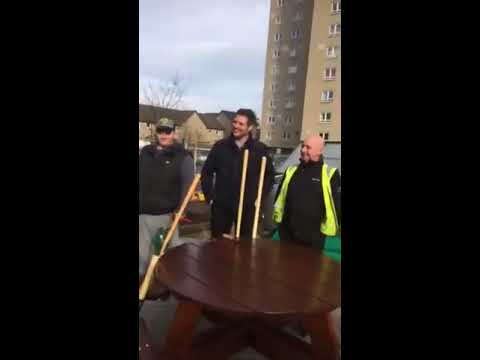This outdoor photograph captures three men standing around a circular dark brown wooden table, each holding long wooden poles. They appear to be chatting and smiling, exuding an overall sense of happiness. The man on the left is wearing gray sweatpants, a navy blue shirt, a dark-colored vest, and a baseball cap. The man in the middle is dressed entirely in dark colors, including black bottoms and a black top. The man on the right is also clad in dark colors but stands out with a neon yellow crossing guard vest over his black jacket. In the background, a high-rise beige-brown building stretches up to the top of the image on the right, while shorter residential houses line the left, with the branches of a leafless tree visible. The sky above is predominantly blue with some clouds.